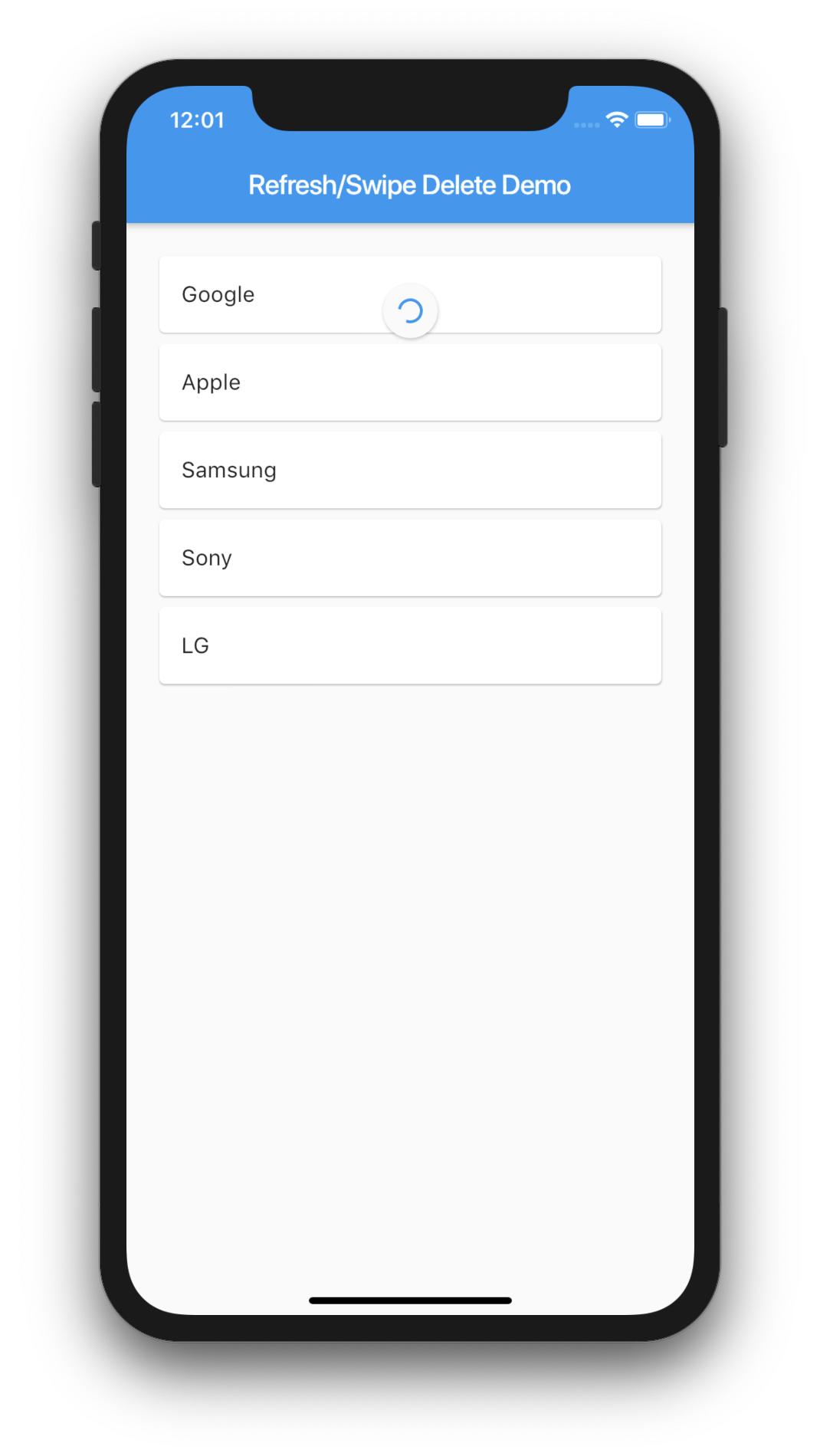This image depicts a cell phone with a black border around its edges. At the center of the screen, the time is prominently displayed as 12:01. On the upper right-hand side, there are three faint dots followed by a Wi-Fi signal icon and a battery indicator. Beneath these indicators, the text "refresh/swipe delete demo" appears in white font inside a blue box that spans the entire width of the top section of the screen. The lower portion of the screen has a white background, displaying five distinct bars, each representing a different brand. From top to bottom, the bars list Google, Apple, Samsung, Sony, and LG. Additionally, a busy icon is situated at the top center of the screen.